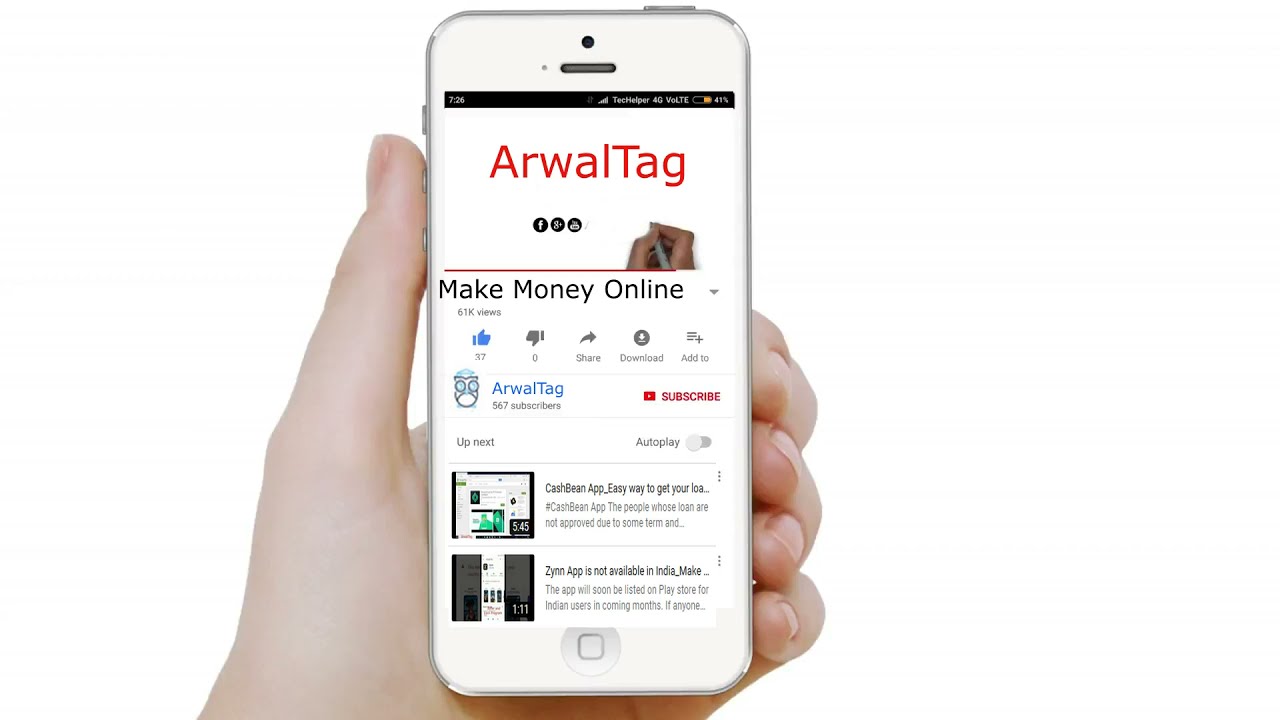The image depicts a white human hand, emerging from the bottom left of the frame, holding a white smartphone with a silver exterior case. The phone is positioned upright with the thumb gripping the left side and the palm supporting the device. The hand and phone are set against a white background.

On the smartphone screen, the time reads 7:26 in the top-left corner with the battery level indicator and 4G status displayed in the top-right. The main display shows a YouTube video in the app, featuring the channel "R-Wall Tag." The video title, written in red letters, is "R-Wall Tag," and beneath it in black lettering is "Make Money Online."

The screen also shows typical YouTube interface elements, such as the like, dislike, share, download, and add-to buttons. There are 37 likes and zero dislikes. Additionally, there are icons for Facebook, Google Plus, and a third unknown icon resembling a radio. Below the video section, a blurred list of recommended videos is barely visible. The presence of various colors including white, red, black, light blue, tan, green, and light brown adds detail to the screen content, highlighting different interface elements and video thumbnails.